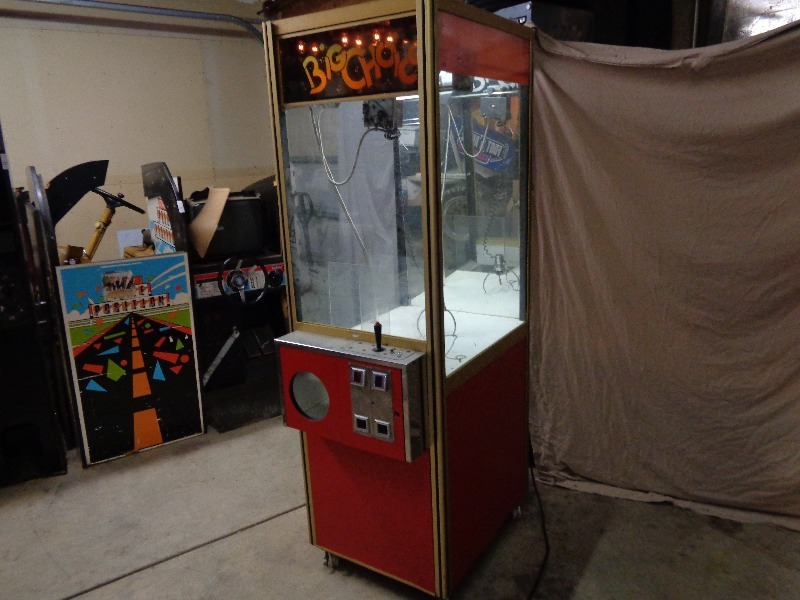This detailed photograph depicts the interior of a cluttered garage-turned-storage unit for arcade equipment. Dominating the foreground on the right is a large, upright rectangular object draped in gray fabric, concealing its contents. Adjacent to this covered object is a disused crane game machine, marked with the title "Big Choice" in bold letters at the top. The red-trimmed machine features an empty clear glass case, its claw perched and inactive on the platform inside, and an operational joystick. Nearby, there are slots for inserting quarters and retrieving prizes, although the machine currently holds none.

Further left, at the very center of the image, lies the detached panel of an arcade racing game, with the visible remnants of a road scene under a sky filled with clouds, scattered with various shapes including triangles, circles, and rectangles. The artwork suggests a whimsical, almost celebratory scene as if a car had driven through confetti. Below the panel, the racing machine's monitor is partially obscured with a piece of cardboard, and the lower portion reveals a steering wheel, gear shift, pedals for acceleration and braking, and part of the cabinet’s seating arrangement. The arcade panel possibly belongs to the adjacent dismantled racing cabinet, indicating it's been taken apart for storage or repair.

On the far left side of the photograph, leaning against unfinished drywall, is a row of various odds and ends, including items in cardboard boxes and miscellaneous bric-a-brac. Also visible is a track for a garage door in the top left corner, emphasizing the setting's initial purpose as a standard garage. The entire scene rests on a concrete floor, and the overall color palette includes muted shades of red, blue, green, orange, white, and gray, contributing to the cluttered yet vibrant chaos typical of storage spaces.